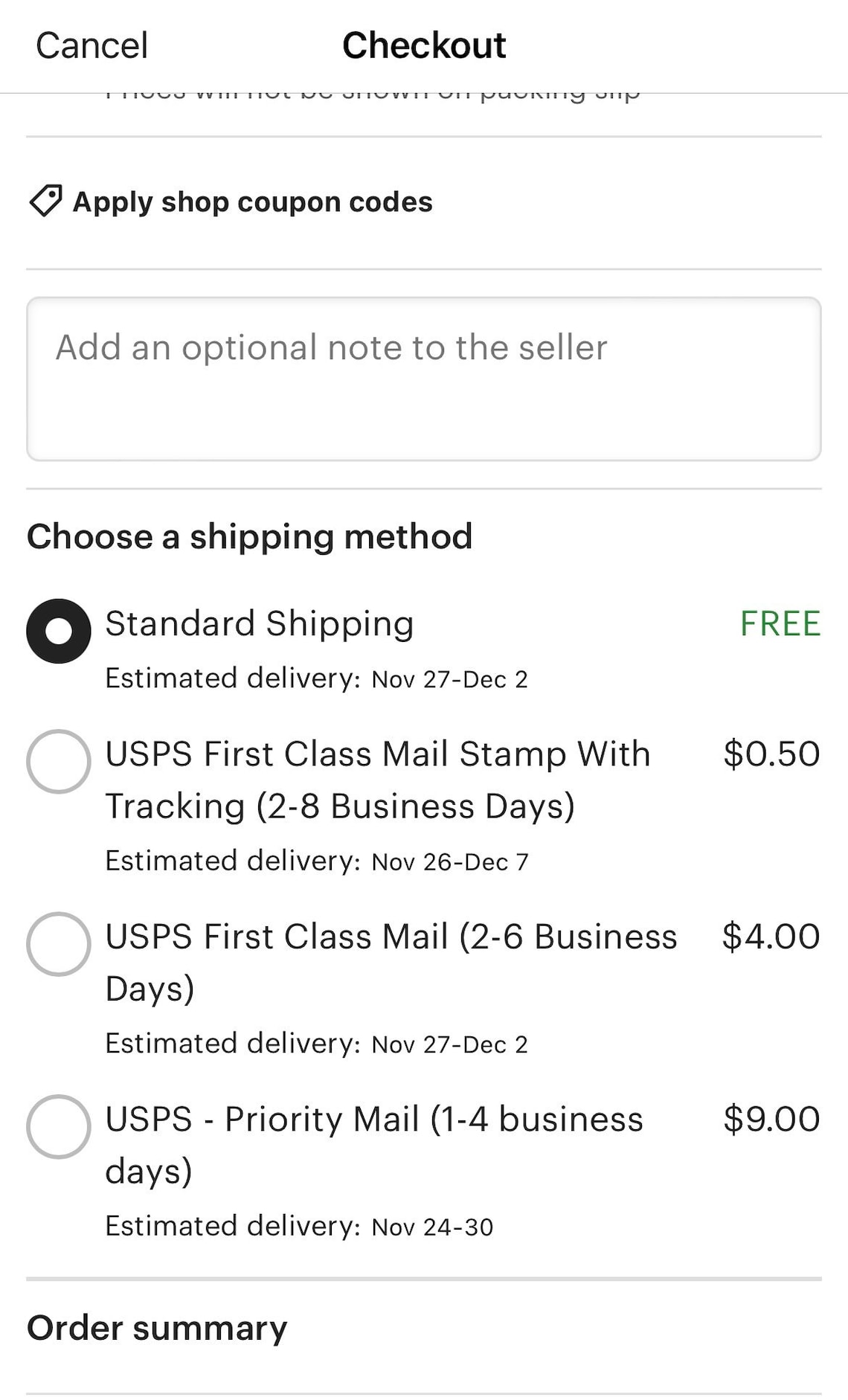The image displays a cell phone screen showcasing a checkout page for product ordering on a white background. At the top left corner, the word "Cancel" is displayed, and next to it, the highlighted word "Checkout" is prominently visible. Below this, a graphic of a price tag accompanied by the text "Apply shop coupon codes" appears. Moving further down, there is a text box with the prompt "Add an optional note to the seller."

The next section is titled "Choose a shipping method" and presents four options, each accompanied by a selectable circle. The circle next to "Standard Shipping" is filled in, indicating it is the selected option, with an estimated delivery date from November 27 to December 1 and the word "FREE" in all caps located across from this option.

The subsequent shipping methods are listed as follows:
1. "USPS First Class Mail (Stamp with Tracking)" with a delivery time of 2-8 business days, estimated delivery between November 26 and December 7, and a fee of $0.50.
2. "USPS First Class Mail" with a delivery time of 2-6 business days, estimated delivery between November 27 and December 2, with a cost of $4.00.
3. "USPS Priority Mail" with a delivery time of 1-4 business days, estimated delivery between November 24 and November 30, for a price of $9.00.

Below the shipping options, a thin dividing line spans the page followed by the text "Order Summary" in a bolder font, marking the end of the visible content on the page.